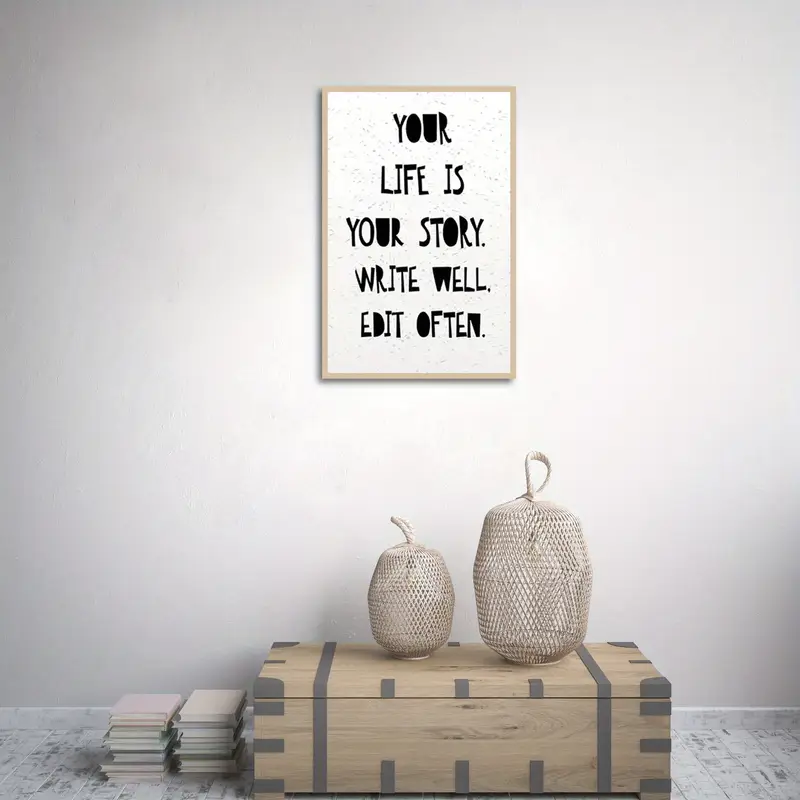The image depicts a framed picture hanging on a wall, featuring an inspirational quote in black text that reads, "Your life is your story. Write well. Edit often." Below the framed picture, a wooden chest serves as the focal point. Positioned atop the chest are two decorative objects crafted from ropes, tied together to form oval shapes. One of these objects is noticeably smaller than the other. These rope decorations appear to be purely ornamental, adding a touch of rustic charm to the room's decor. At the base of the chest, there is a neat stack of pale-colored books, contributing to the cozy and inviting atmosphere.